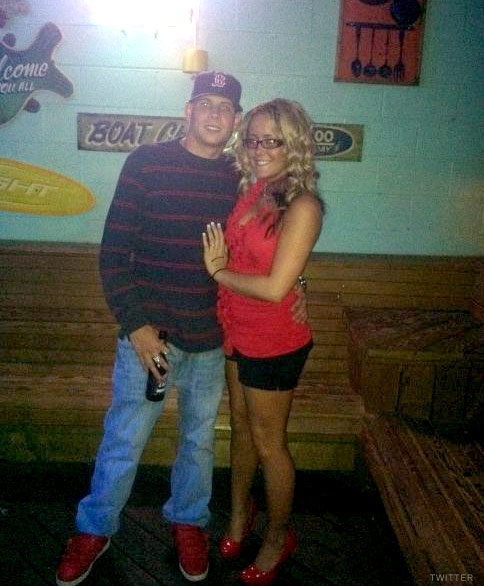The image features a young couple, possibly in their 20s, standing in what appears to be a bar or a casual dining area. The woman on the right has long, curly blonde hair and is wearing glasses, a red (or pink) shirt, black shorts, and red shoes. She has her hand on the chest of the man beside her. The man on the left is wearing a blue and red striped sweater, blue jeans, red shoes, and a dark blue Boston Red Sox cap. He has his arm around the woman and is holding a glass beer bottle.

They stand in front of a blue cinder block wall with a window letting in some light. The background also features wooden benches that run along both the back and side walls of the corner, adorned with various pictures and signs. One sign has the word "boat" on a gray background with blue letters. Another sign reads "welcome" in white letters on a green background, and there's a third sign with light letters on a yellow background, which is partially obscured. There's also a picture of spoons and ladles on an orange background. A light fixture illuminates the scene from above. The overall ambiance suggests a cozy, casual bar setting.